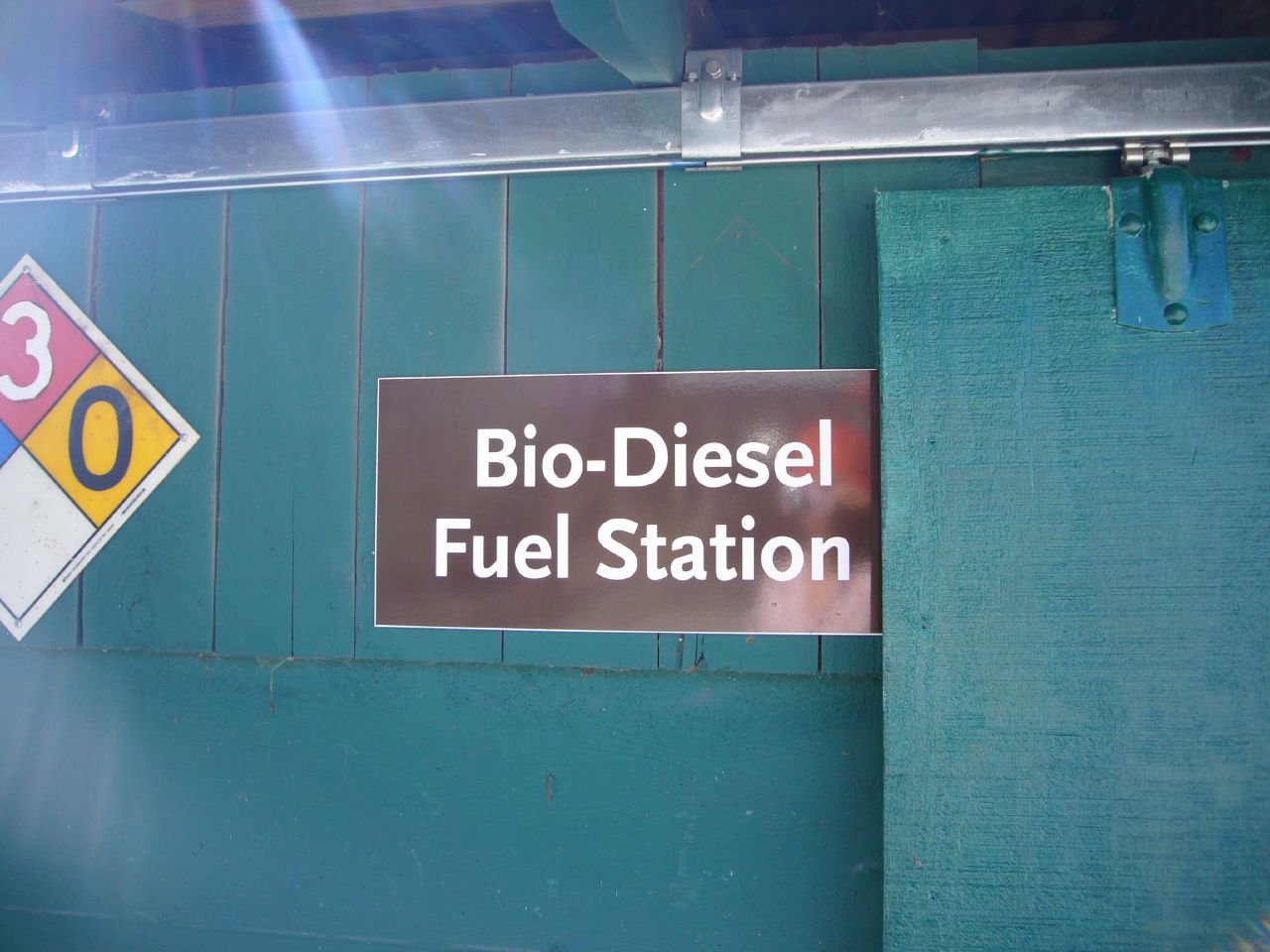The color photograph features a teal wooden wall adorned with various signs and fixtures. Centrally located on the wall is a rectangular, brown sign with white lettering that reads "Biodiesel Fuel Station." To the left of this sign is a diamond-shaped hazard sign, outlined in white and tilted at a 45-degree angle. The visible sections of this hazard sign include a white number three on a red background and a black zero on a yellow background. At the top of the wall, a silver metal bar runs horizontally from left to right, providing support for a wooden door that matches the teal color of the wall. A blue latch is visible on this door.